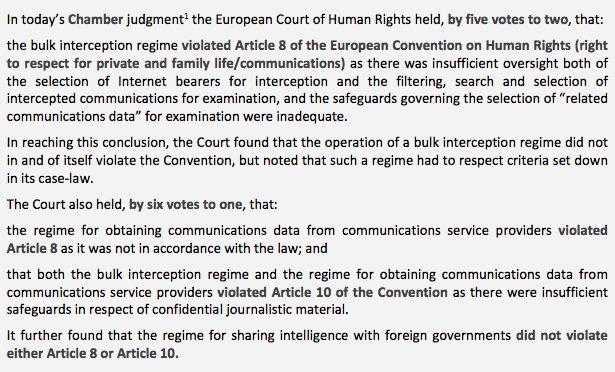The image displays a light gray screen resembling a computer monitor. The screen features black text detailing a judgment from the European Court of Human Rights. The judgment is structured in several paragraphs, each elucidating critical aspects of the decision:

1. **Introduction**: The European Court of Human Rights ruled by a majority of five votes to two that the bulk interception regime violated Article 8 of the European Convention on Human Rights, which protects the right to respect for private and family life, including communications. The court cited insufficient oversight in both the selection of internet bearers for interception and the filtering, searching, and selection of intercepted communications, as well as inadequate safeguards for examining related communications data.

2. **Findings**: The court concluded that while the operation of the bulk interception regime itself did not violate the Constitution, it must adhere to criteria established in case law to ensure compliance with human rights standards.

3. **Additional Violations**: The regime for obtaining communications data from service providers also violated Article 8 by not being in accordance with the law. This decision was reached by a majority of six votes to one.

4. **Article 10 Violation**: Both the bulk interception regime and the regime for obtaining communications data from service providers were found to violate Article 10 of the Convention, which protects freedom of expression and information.

The screen contains no additional elements or decorations, focusing solely on the detailed judgment text.